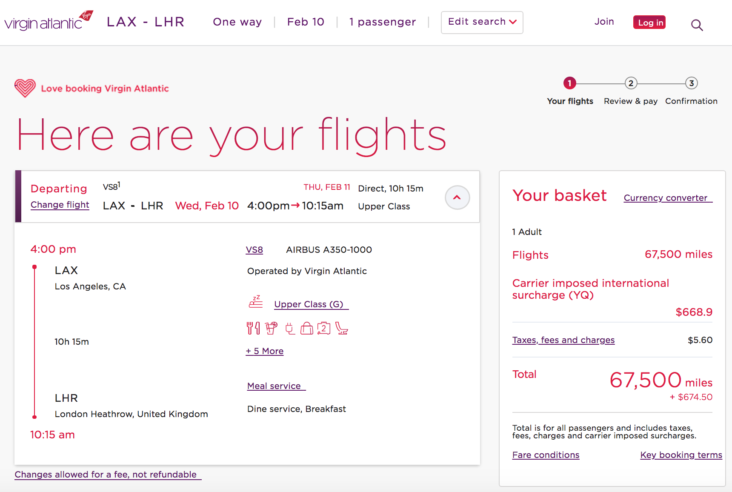This screenshot captures a detailed view of a flight booking website, specifically Virgin Atlantic, for a one-way trip from Los Angeles International Airport (LAX) to London Heathrow Airport (LHR) on February 10th. The user is booking for one passenger, with the option to edit their search. At the top right corner, navigation options include "Join," "Login," and a search icon (magnifying glass).

The booking process is divided into three steps: "Your Flights," "Review and Pay," and "Confirmation." The user is currently on step one, indicated by the number one highlighted in red.

The flight details show a direct departure from LAX to LHR on Wednesday, February 10th at 4:00 PM, arriving at 10:15 AM on Thursday, February 11th. The flight duration is 10 hours and 15 minutes in Upper Class. There is a dropdown tab providing further details: departure at 4:00 PM from LAX, and landing at LHR at 10:15 AM on an Airbus A350-1000, flight number VS8, operated by Virgin Atlantic. The flight amenities include icons for food, drinks, power outlets, baggage, and seating, with an additional five amenities accessible via a clickable tab. Meal service options such as dine service and breakfast are also provided for user preferences.

On the right side of the screenshot, a large rectangle labeled "Your Basket" includes a currency converter feature. The basket shows the cost breakdown: 67,500 miles for one adult flight, with a carrier-imposed international surcharge (YQ) of $668.90, taxes, fees, and charges amounting to $5.60, making the total cost 67,500 miles plus $674.50. The total includes all taxes, fees, charges, and surcharges.